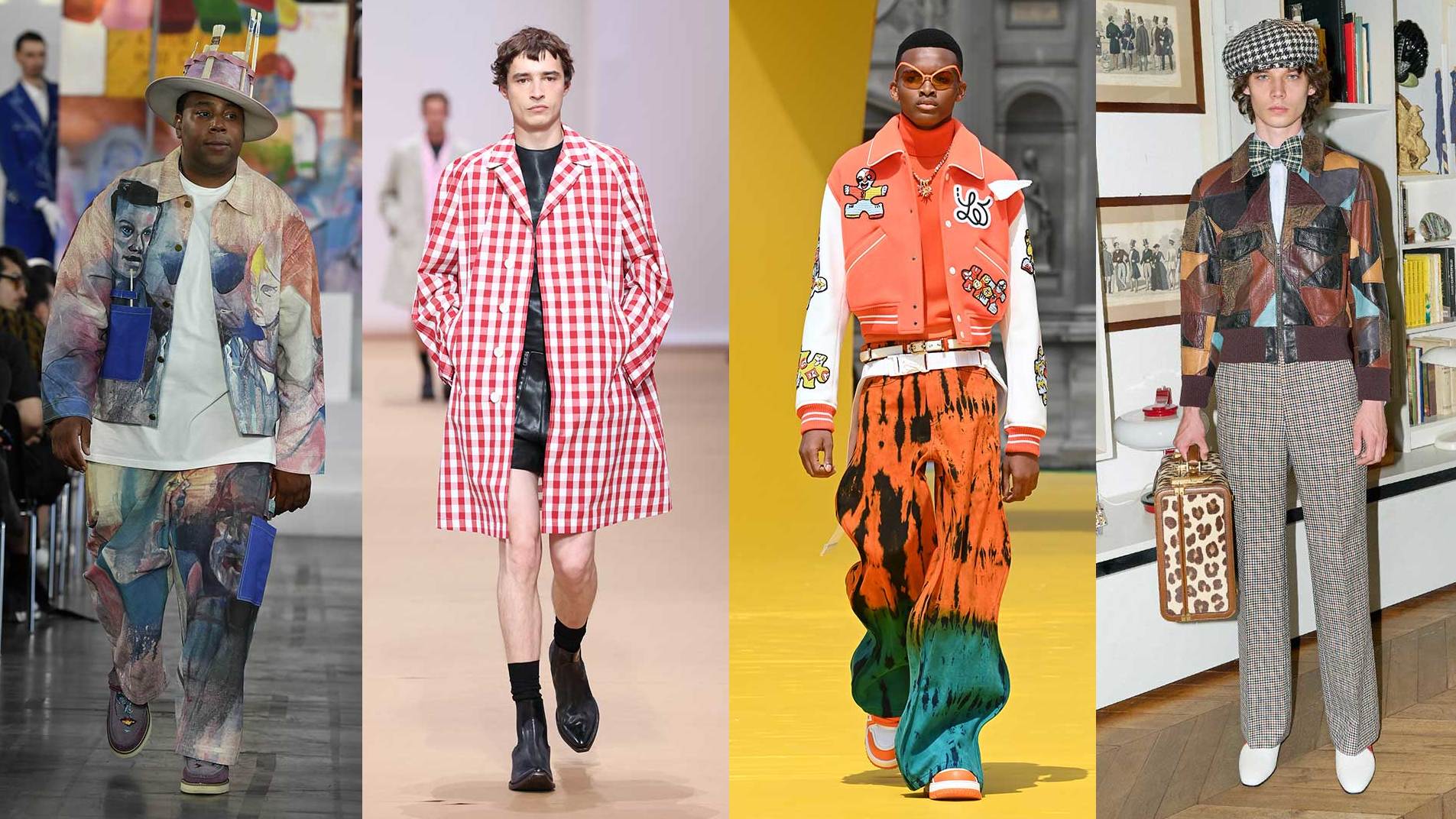This image is a collage of four individual photos featuring four men dressed in high-fashion outfits that showcase bold and eclectic styles. 

Starting from the left, the first individual appears to be Kenan Thompson from Saturday Night Live, walking on a colorful runway with spectators in the background. He is wearing a multicolored suit with pastel shades of blue, pink, and white, adorned with faces and abstract designs. Accompanied by a white t-shirt, he also sports white gloves, grey shoes, and a distinct pink hat with brush-like attachments.

The second panel features a Caucasian male walking on a brown-floored runway with a gray background. He dons a red and white checkered overcoat paired with shiny black shorts. His look is completed with black socks and boots. The model's hands are in his pockets, adding a casual flair to his striking outfit.

In the third panel, we have a black male model striding down a yellow runway framed by architectural designs. He is wearing vibrant, loose-fit tie-dye pants in orange, green, and black, paired with white and orange shoes. His orange and white letterman-style jacket with cartoon emblems is striking, complemented by an orange high-neck shirt, white belt, funky orange sunglasses, and a necklace.

Finally, the rightmost image shows a young white male standing in a room with wooden flooring and a background filled with photo frames and bookshelves. He is dressed in a vintage patchwork leather jacket made from various colors like black, brown, gray, yellow, and blue. He pairs this with pleated pants, white boots, a white shirt with a bow tie, and a checked beret hat. His look is accessorized with a leopard print briefcase.

This fashion collage excellently captures a spectrum of creative and avant-garde styles.